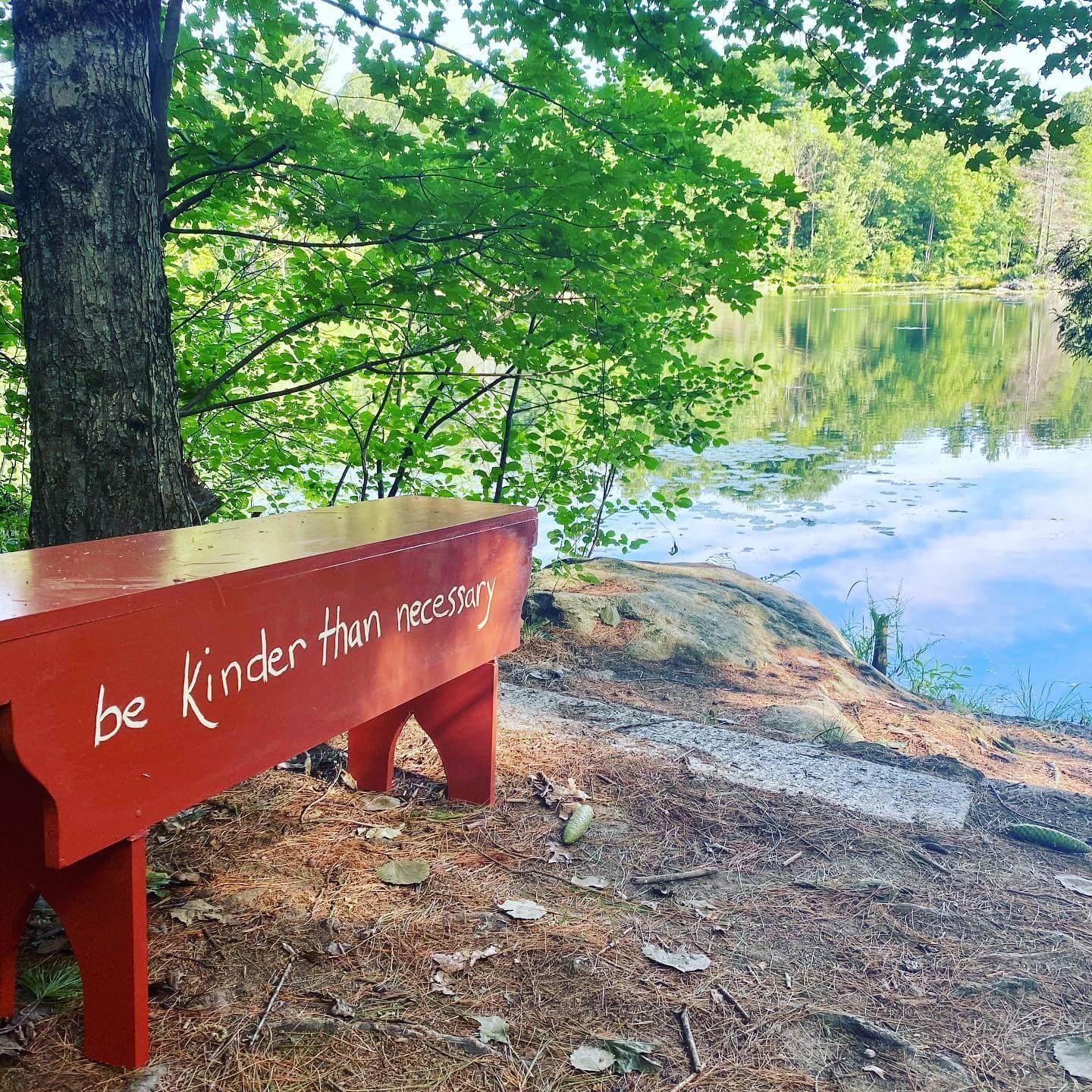This photograph, set within a rectangular frame, captures a peaceful outdoor nature scene in vivid detail. Dominating the left-center of the image is a carved and painted red wooden bench standing on connected legs, with an artful cutout design at the bottom. Hanging from the top surface of the bench is a sign featuring the inspirational quote, "be kinder than necessary," in white, handwritten-style lowercase letters. The foreground reveals a dirt slope with scattered bark and leaves, leading to a calm body of water centered in the image. This reflective pond, tinged with blue and marked by gentle ripples, mirrors the trees standing along its far edge. To the upper middle and right of the photograph, various tree trunks and foliage frame the scene, with a notable gray tree trunk on the left and green leaves against a blue sky in the backdrop. A dead, gray tree can also be seen on the far right. The overall setting suggests a tranquil day in nature, making it suitable for a calendar of scenic landscapes and inspirational messages.